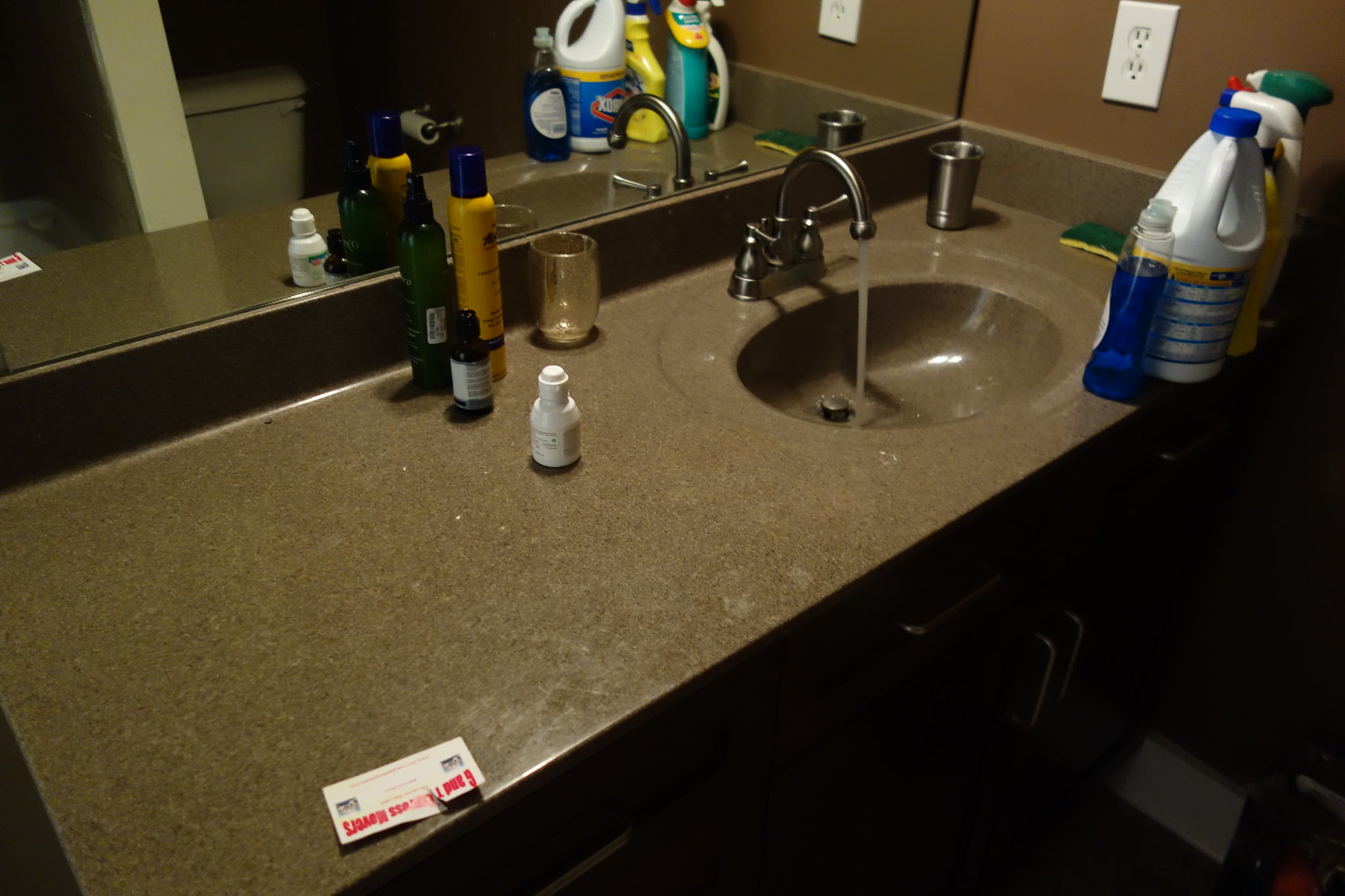In this photograph, a well-used bathroom sink is captured in detail. The sink's continuous brown, mottled stone countertop complements the brushed nickel fixtures, with the faucet turned on and the left handle extended outward. Various toiletry items, including a silver cup, a cleaning pad or brush, and a mix of cleaning products, are scattered around the sink. The cleaning products consist of a small bottle of contact lens solution, a bottle of hair product spray, a small brown bottle, a green bottle, a larger bottle of bleach, cleaning spray, and dish soap. The counter is adorned with a white outlet, contrasting with the brown painted wall behind it. A large mirror runs the length of the bathroom counter, reflecting the top tank of a toilet and a partial view of a bathtub separated by a dividing wall. The room appears dimly lit, adding to the overall moodiness of the scene. A torn business card can be seen at the far edge of the counter, away from the cluster of cleaning items.